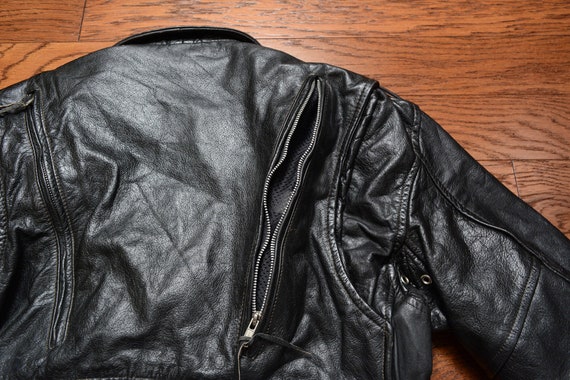This square, full-color photograph, taken indoors under artificial light, captures a detailed close-up of the back of a black leather jacket laid out on a dark brown, stained wooden table or countertop. The leather jacket features two zippers running diagonally from the shoulders to the mid-back. The zipper on the right is fully unzipped, revealing a mesh lining underneath designed for breathability, while the zipper on the left is zipped up and closed. The image includes visible portions of the right sleeve extending outward but does not show the left sleeve. The jacket's placement and the careful emphasis on the zippers suggest the photo may have been taken to showcase these specific details, possibly for an online sale listing.